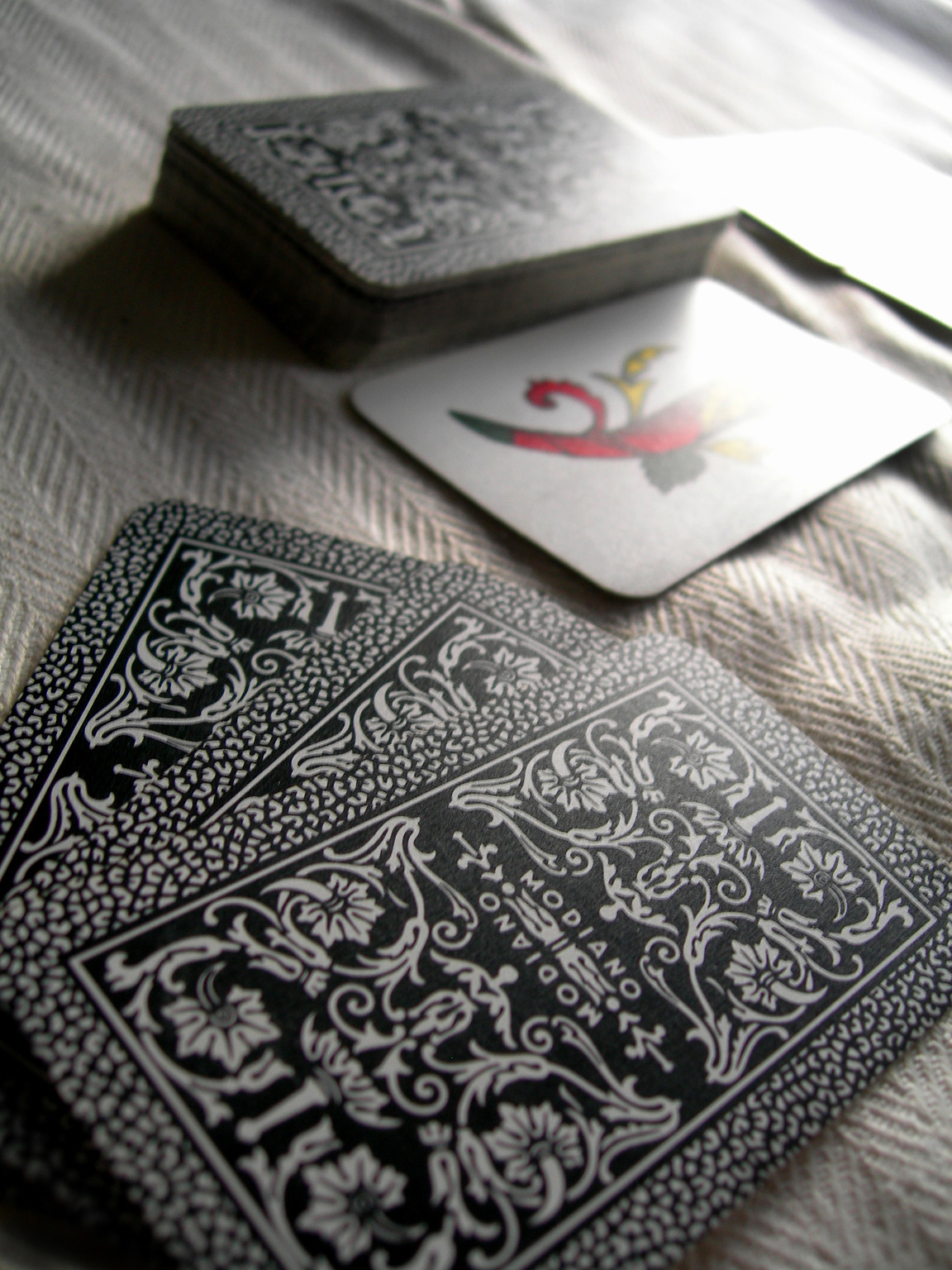The image depicts a deck of cards placed on a soft, grey and white surface that resembles a blanket with a smooth texture. The deck is arranged in a single stack. To the right of the stack, a single card is face-up, featuring a character in red, yellow, and black. However, the image clarity is compromised by a large white glare that obscures half of the card, making it difficult to determine specific details; it appears similar to a joker card. Below it, three cards are face-down, showcasing the intricate floral-like patterns on the card backs, which are colored in black and white. The design features the word "Modano" at the center and a border composed of small white U-shaped patterns set against a black background.